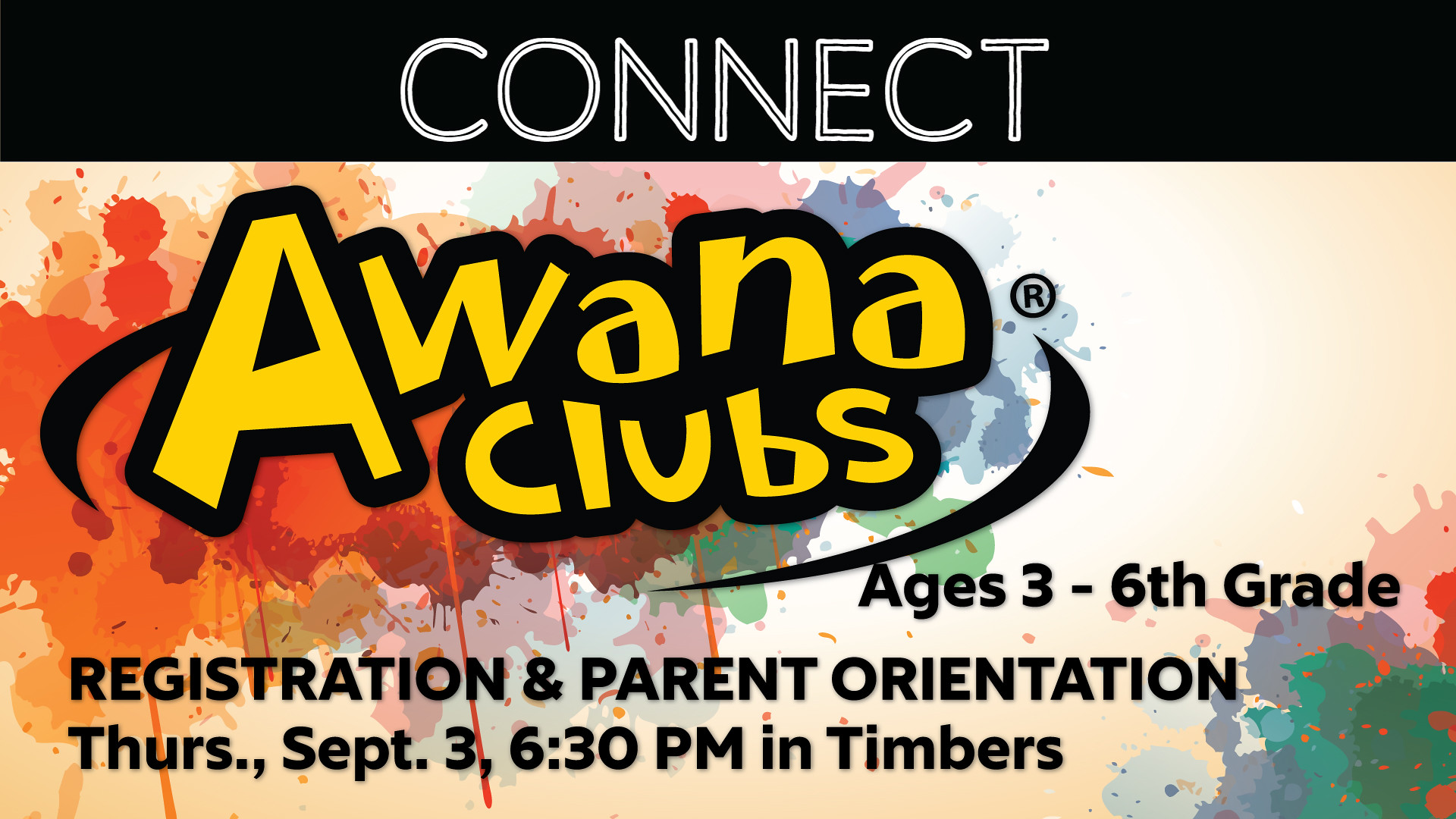This advertisement features a dynamic design with prominent elements and colorful aesthetics. At the top, a black horizontal bar spans the width of the image, displaying the word "CONNECT" in bold white letters. Below, the background resembles a parchment-colored canvas splattered with vibrant paint splotches in an array of colors including orange, yellow, blue, green, tan, red, purple, and light blue, giving a playful and lively effect.

The focal point of the ad is the "AWANA CLUBS" logo, showcased in large, bold yellow letters with a thick black outline. The text is encircled by black crescent shapes, reminiscent of a swish or swoosh, similar to the Nike logo, which enhances the dynamic feel of the design.

Underneath the "AWANA CLUBS" logo, in black letters, it states, "AGES 3 to 6th grade." Further down, also in black, it reads, "REGISTRATION AND PARENT ORIENTATION," followed by the event details, "THURSDAY, SEPTEMBER 3, 6:30 PM IN TIMBERS." The varied paint splotches extend to the edges of the image, with a concentration of green, blue, red, and light blue splashes at the lower right corner, providing a balanced and eye-catching visual appeal.